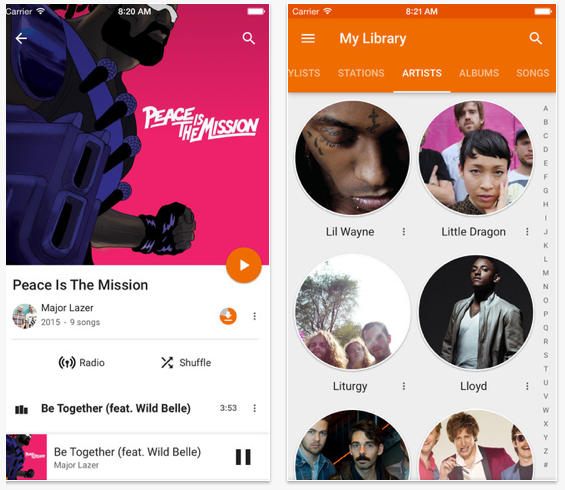The image consists of two screenshots taken from a phone. The left screenshot displays a music player interface. At the top, there is cover art for a song featuring a dark-skinned man with a beard, wearing white sunglasses and a blue tactical vest, set against a hot pink background. To the middle right of the man, the text "Peace is the Mission" appears in white. Below the cover art, the same phrase, "Peace is the Mission," is repeated in black text over a white section. An orange play button with a white triangle is positioned to the right of the title. Immediately beneath, additional details state: "Mazer Lazer 2015" and "nine songs." Directly below this, radio and shuffle buttons are displayed side by side.